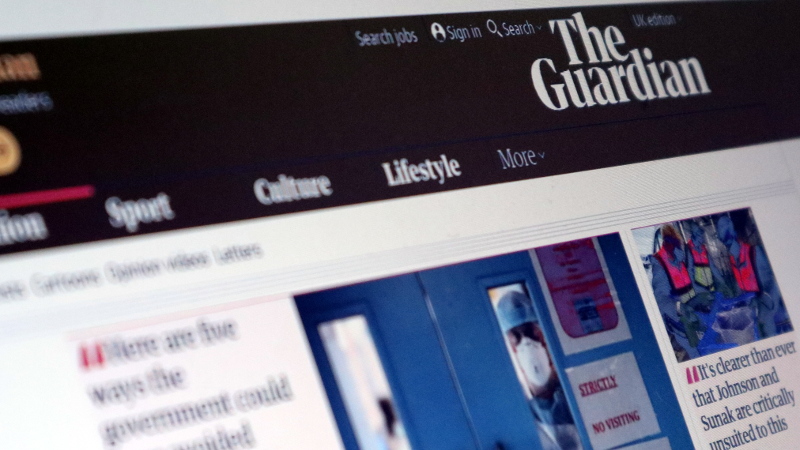The image depicts a slightly angled and partially blurred photograph of The Guardian's website displayed on a screen. The blurriness increases toward the left side, which is closer to the viewer. The Guardian's logo is centrally positioned at the top, accompanied by options such as "Search jobs," "Sign in," "Search," and "UK edition" towards the right. A navigation menu below lists categories including Sport, Culture, Lifestyle, and a dropdown for more options.

The header image features a man clad in medical attire, including a blue coat or robe and a protective cap, standing behind doors with visible warning signs. He is also wearing a face mask, indicative of a medical or hazardous environment. To the right of this central image, there is another photo depicting workers, possibly engaged in trash collection or similar activities.